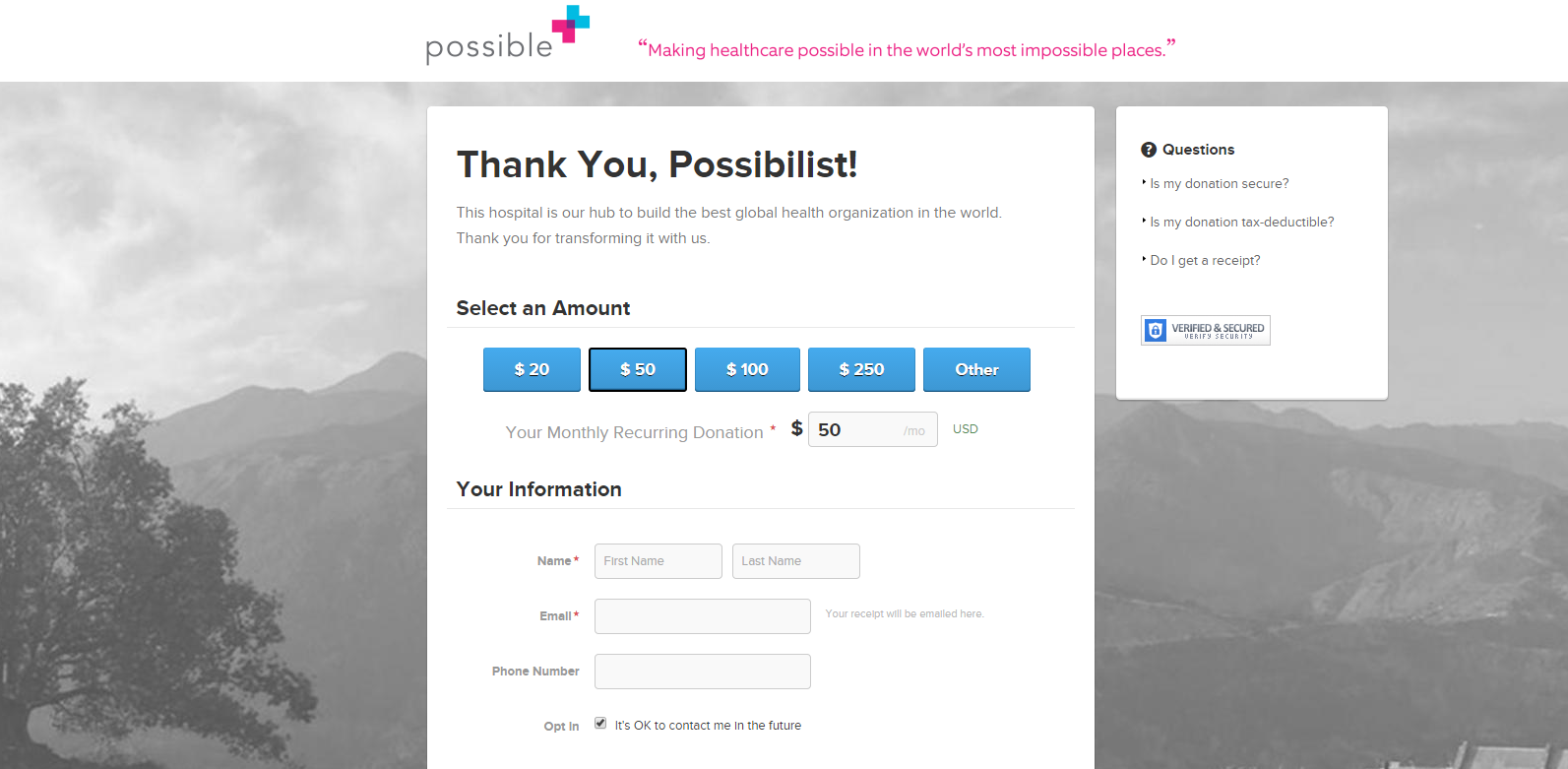In the image, the word "Possible" is prominently displayed at the top. Adjacent to the upper right corner of this word is an icon resembling a plus sign, with its left half in blue and the right half in a purple-pink hue. Next to "Possible," there is a quote in pink lettering that reads, "Making health care possible in the world's most impossible places."

Below this, there appears to be a form for user input, accompanied by a message that says, "Thank you, Possible List. This hospital is our hub to build the best global health organization in the world. Thank you for transforming it with us." Beneath the message, users are prompted to "Select an Amount," with preset options of $20, $50 (which is currently highlighted), $100, and $250, as well as an option for "Other." Further down are fields for personal information such as name, last name, email, and phone number, along with an opt-in checkbox that states, "It's OK to contact me in the future."

The background features a scenic view with mountainous regions and a tree to the right. To the right side of the form, there are frequently asked questions regarding the donation process, including questions like, "Is my donation secure?", "Is my donation tax deductible?", and "Do I get receipts?"

Overall, the image depicts a donation page for a health care organization, with a user preparing to donate $50 to the cause.